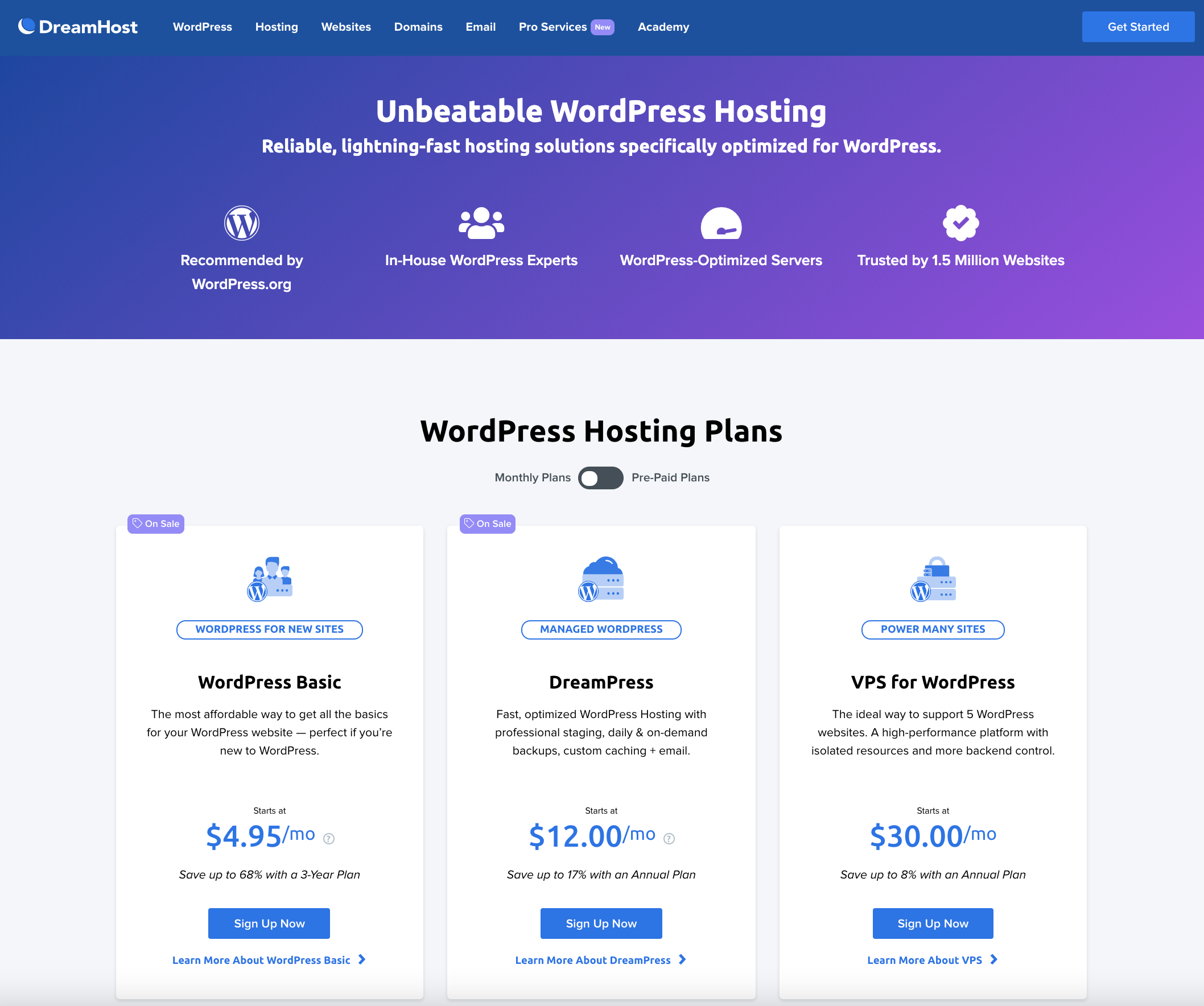This is a screenshot of the DreamHost website, prominently featuring their WordPress hosting offerings. In the top left corner, the DreamHost logo is visible, characterized by a blue circle enclosing a white crescent moon. At the very top of the page, there are seven navigation tabs labeled: WordPress, Hosting, Websites, Domains, Email, Pro Services, and Academy.

The page's main banner showcases a few lines of promotional text: "Unbeatable WordPress Hosting. Reliable, lightning-fast hosting solutions specifically optimized for WordPress." Below this banner, there is a menu displaying three different hosting plans, each presented on a rectangular, portrait-oriented panel.

From left to right, the hosting plans increase in both price and features: 
1. The Basic plan is priced at $4.95 per month.
2. The DreamPress plan costs $12 per month.
3. The VPS for WordPress plan is available for $30 per month.

Additionally, users have the option to choose between monthly plans or prepaid plans, offering flexibility in billing preferences.